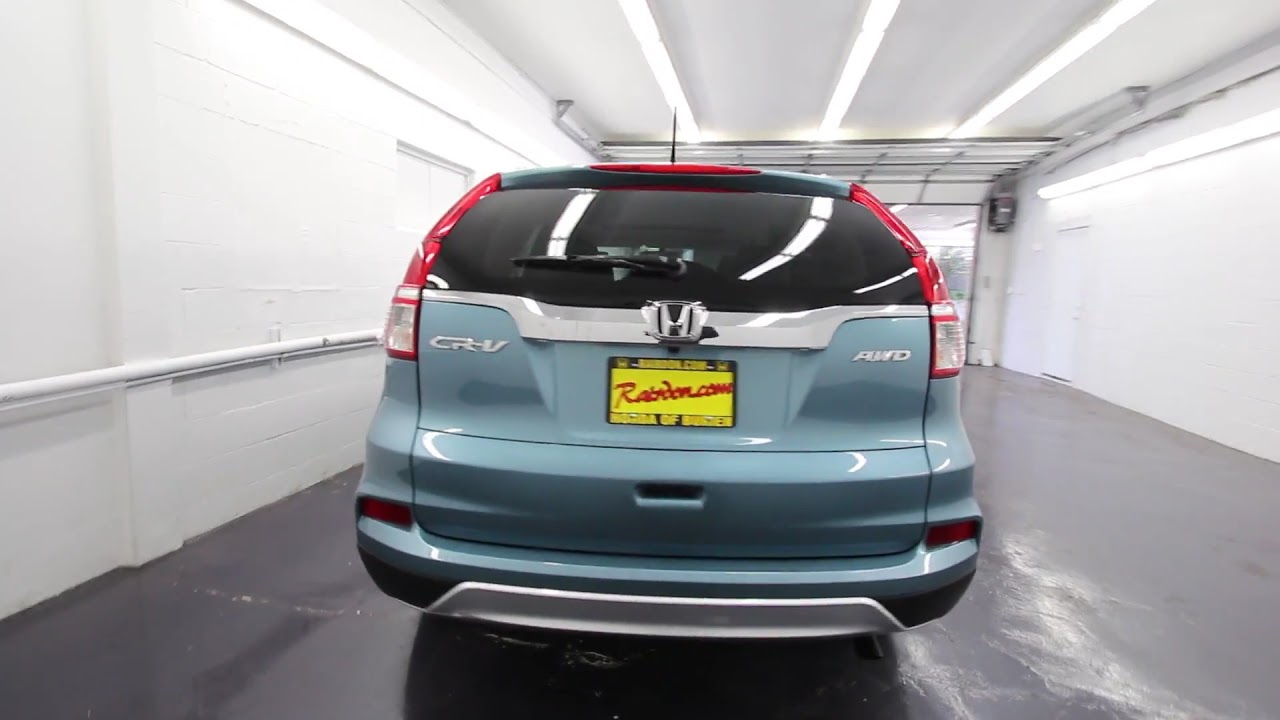This is a horizontally aligned rectangular photograph taken inside a garage, focusing on the back of a new blue Honda CRV. The vehicle prominently displays a black-tinted rear window with a windshield wiper. On the left side of the car, "CRV" is visible, while the right side reads "AWD," indicating it has all-wheel drive. The central logo features the iconic "H" for Honda. The license plate is a temporary yellow paper style with red writing, possibly reading "rabdon.com," although it's slightly blurred, suggesting the person taking the photo may have been moving. The garage itself has bare white cinder block walls, a white ceiling with long fluorescent lights, and a very clean, dark gray cement floor. The garage door is open, revealing a glimpse of distant trees.